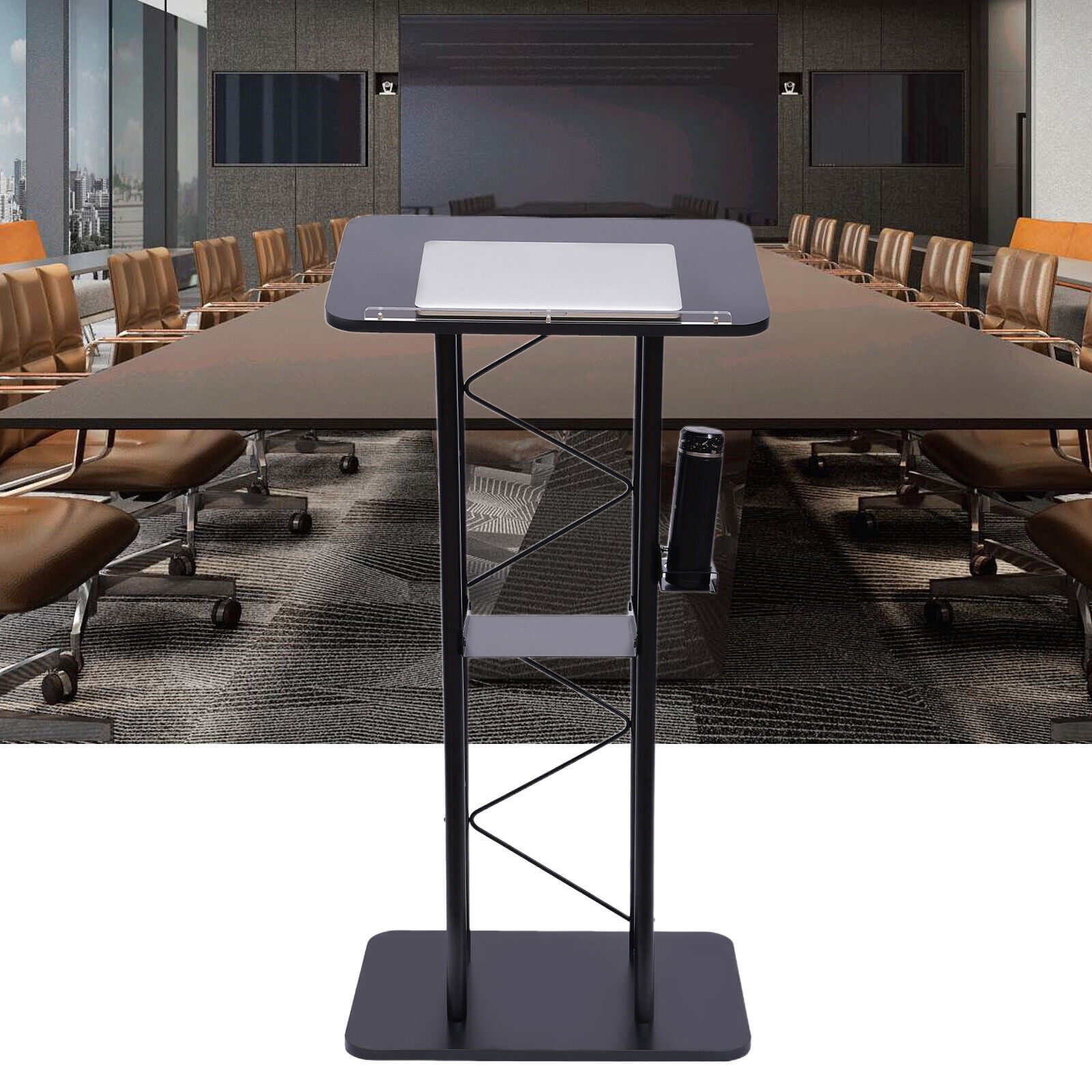This image features a modern, black podium with a sleek, zigzagging support structure cascading down the center, standing on a rectangular base. A closed silver laptop rests on the black top of the podium. It appears to be superimposed over the foreground of a conference room. The room itself is spacious, with a large, wide brown table surrounded by numerous light brown office chairs, likely leather, offering seating on both sides. The room has a neutral-colored carpet with gray and brown swirly stripe patterns. The back wall features a massive, shiny black screen for presentations, flanked by two smaller screens on either side. Vertical glass windows on the right side allow views of surrounding cityscape, with buildings and a blue sky in sight. Small hints of orange suggest the presence of couches, adding a pop of color to the professional setting.